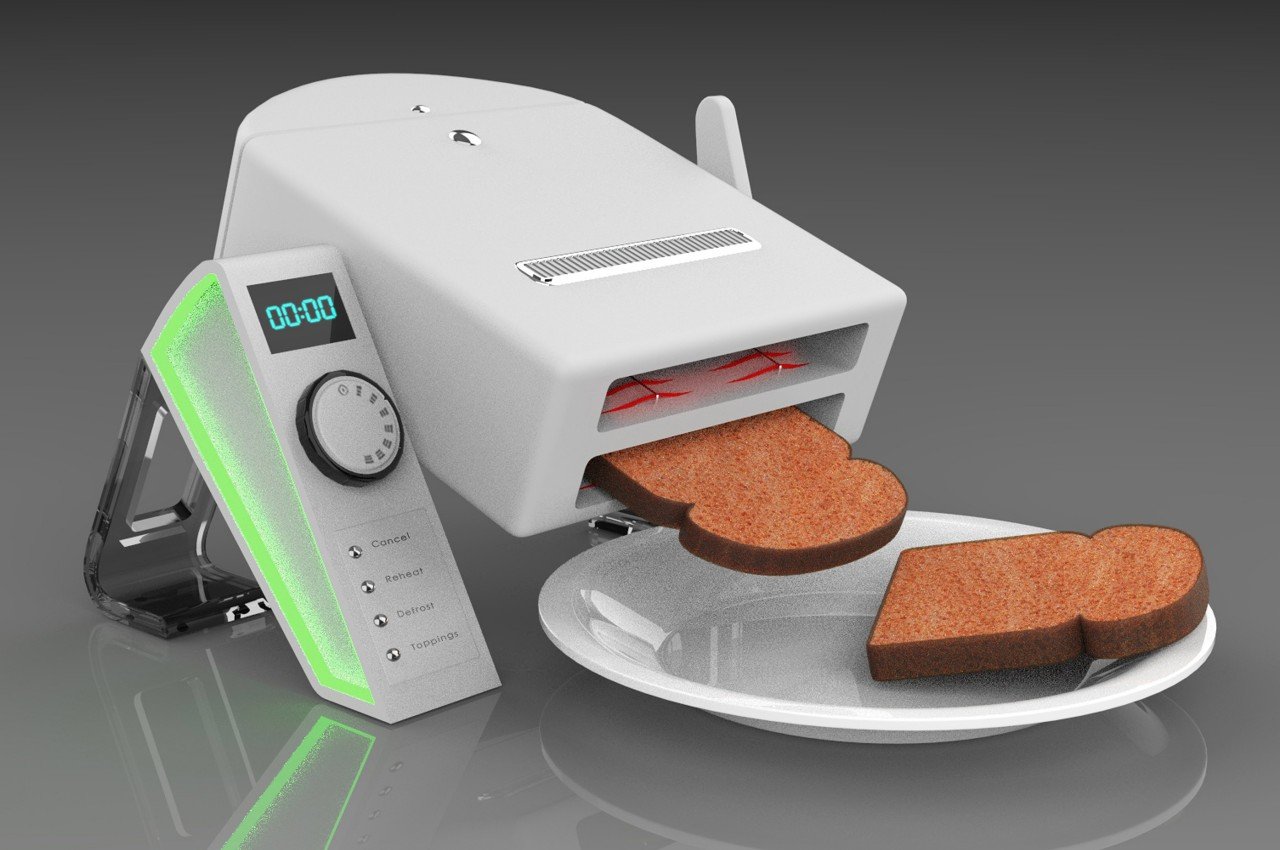This image showcases a modern, innovative toaster with a unique, slanted design. The toaster is predominantly white with a square shape and a rounded back. It features two slots: one on top, which appears to have red heating elements visible, indicating where the bread is toasted, and another slot at the bottom where the toast emerges. The toaster is placed to the left of a white round plate that catches the toast as it slides out. The entire setup gives a sense of a streamlined and efficient toasting process. Adjacent to the toaster, there's a round dial with numbers on it, likely for adjusting the toast's browning level, and above this dial is a small digital screen that appears to display a timer. The background is a muted, empty gray, emphasizing the toaster and its functionality. The colors in the image include neon lime green, white, red, toasty brown, brown, black, and gray, giving it a futuristic yet cozy feel. The toast itself appears very bright and slightly unrealistic, suggesting it may have been digitally enhanced.